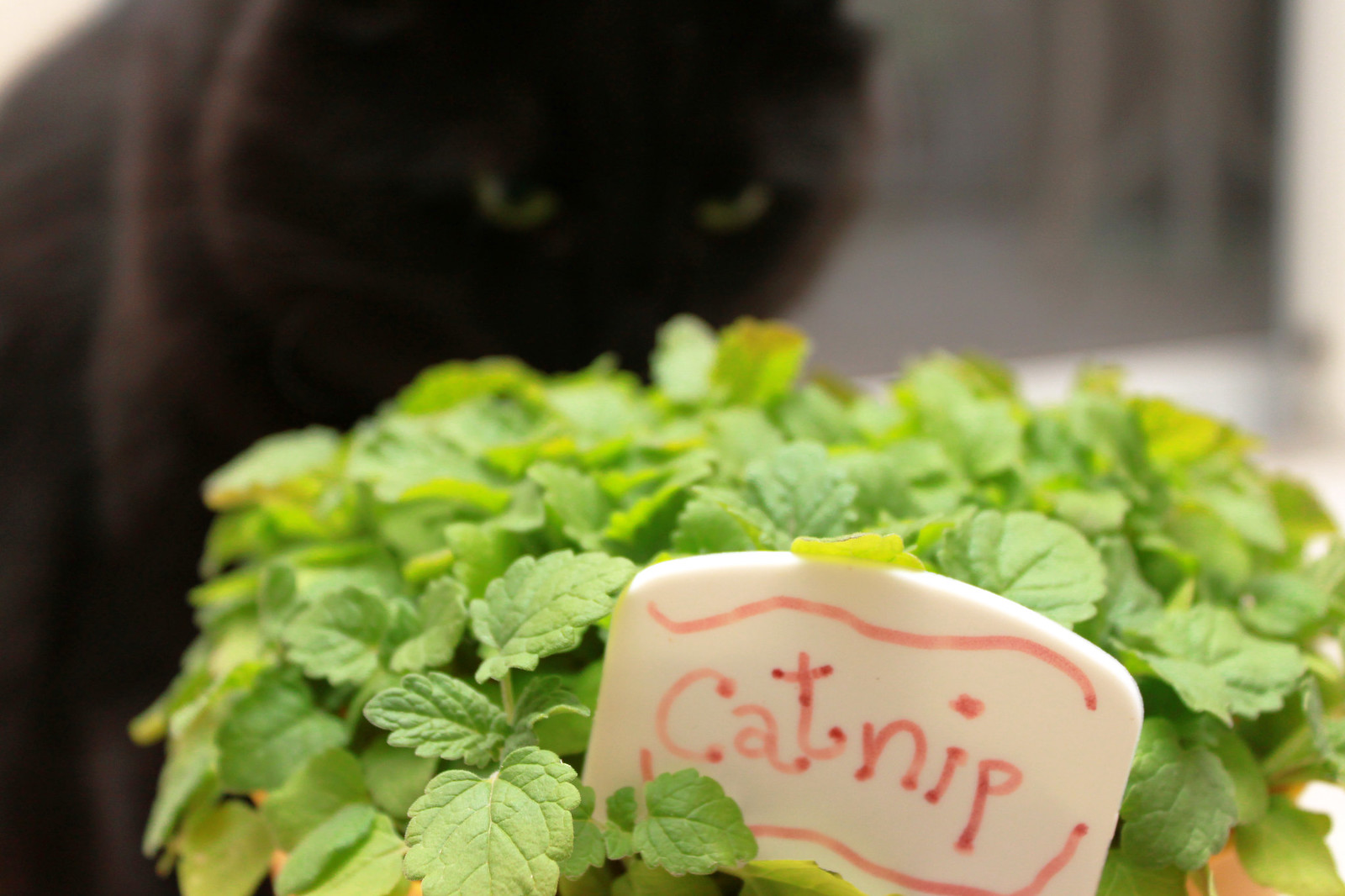In this photo, a windowsill frames a household scene where a pot of fresh, low-growing catnip takes center stage. The catnip, identifiable by its serrated leaves, is labeled with a white name tag marked in red ink, featuring a distinct swirl design above and below the word "catnip." In the blurry background, a large black cat with striking green eyes fixates on the plant, seemingly eager to investigate or nibble on it. The softly blurred window and surrounding elements accentuate the focus on the cat and the thriving catnip, highlighting a serene domestic moment.